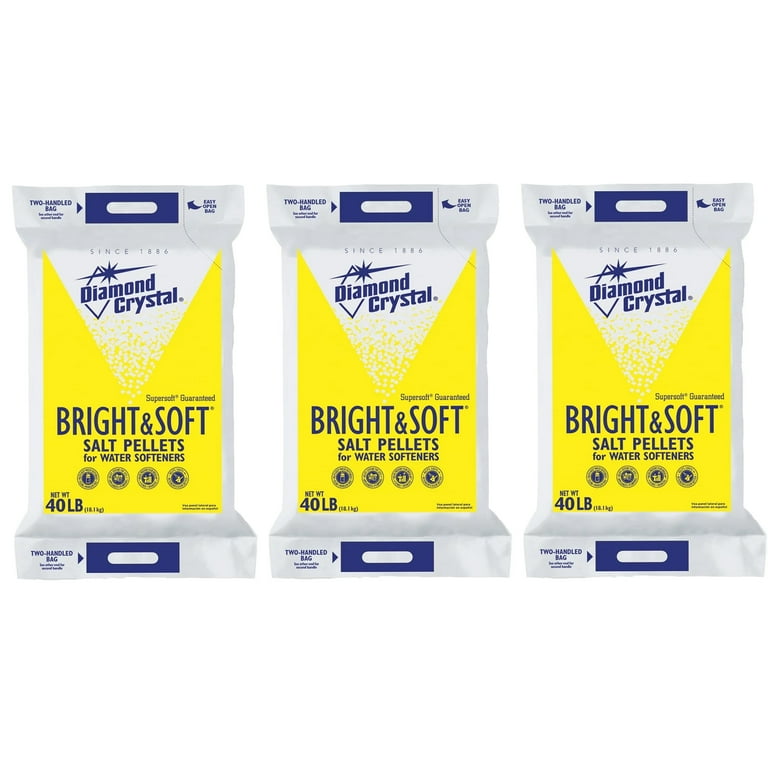The image features three Diamond Crystal Bright and Soft Salt Pellets bags for water softeners, arranged flatly side-by-side against a white background. Each 40-pound bag is predominantly white with a prominent yellow vertical rectangle in the middle, accented by blue lettering. The yellow rectangle features the product name: "bright and soft salt pellets for water softeners," along with a white triangle at the top that transitions from solid white to a salt crystal appearance, containing the Diamond Crystal brand name. The bags have practical two-handled designs for easy carrying, highlighted by a sign at the top showing an arrow pointing to "empty bag." Additional symbols and writing are present but not fully legible in the image.